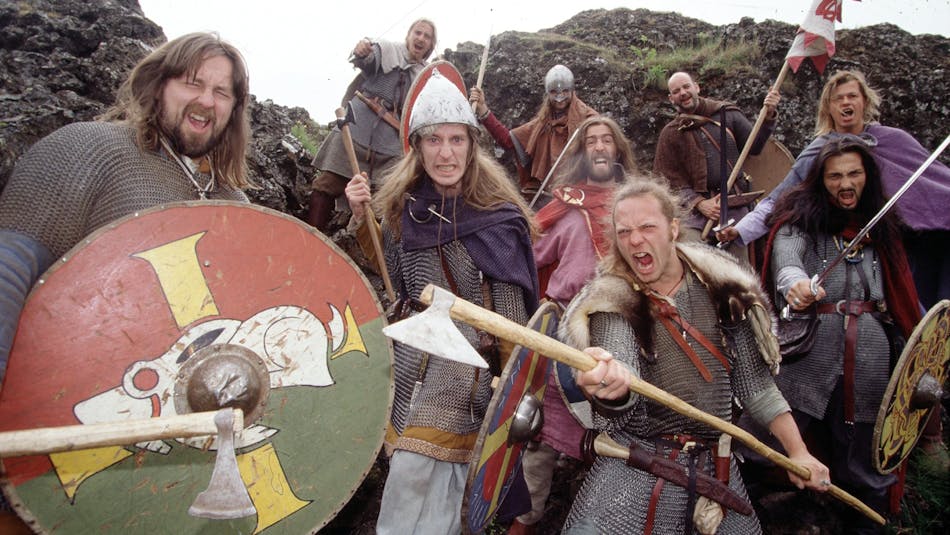The horizontally aligned rectangular image captures a group of ten men dressed in medieval Viking attire, standing outdoors on what appears to be a jagged, uneven slope or possibly a hilltop. Their expressions range from fierce to stoic as they face the camera, suggesting they might be participating in a historical reenactment or festival. Dominating the left side, a man stands in the foreground holding a large circular shield, split into red and green halves, adorned with a yellow cross and intricate decoration, alongside an axe. The rest of the group, arrayed to his right, brandish various weapons, primarily long wooden rods with axe heads, and wear armor. Only two among them wear helmets: the man right behind the shield bearer, and another in the center-back whose helmet partially obscures his face. Their hair colors vary from blonde to black. The background features large, dark brown rock structures with patches of green grass and moss, under a white sky.